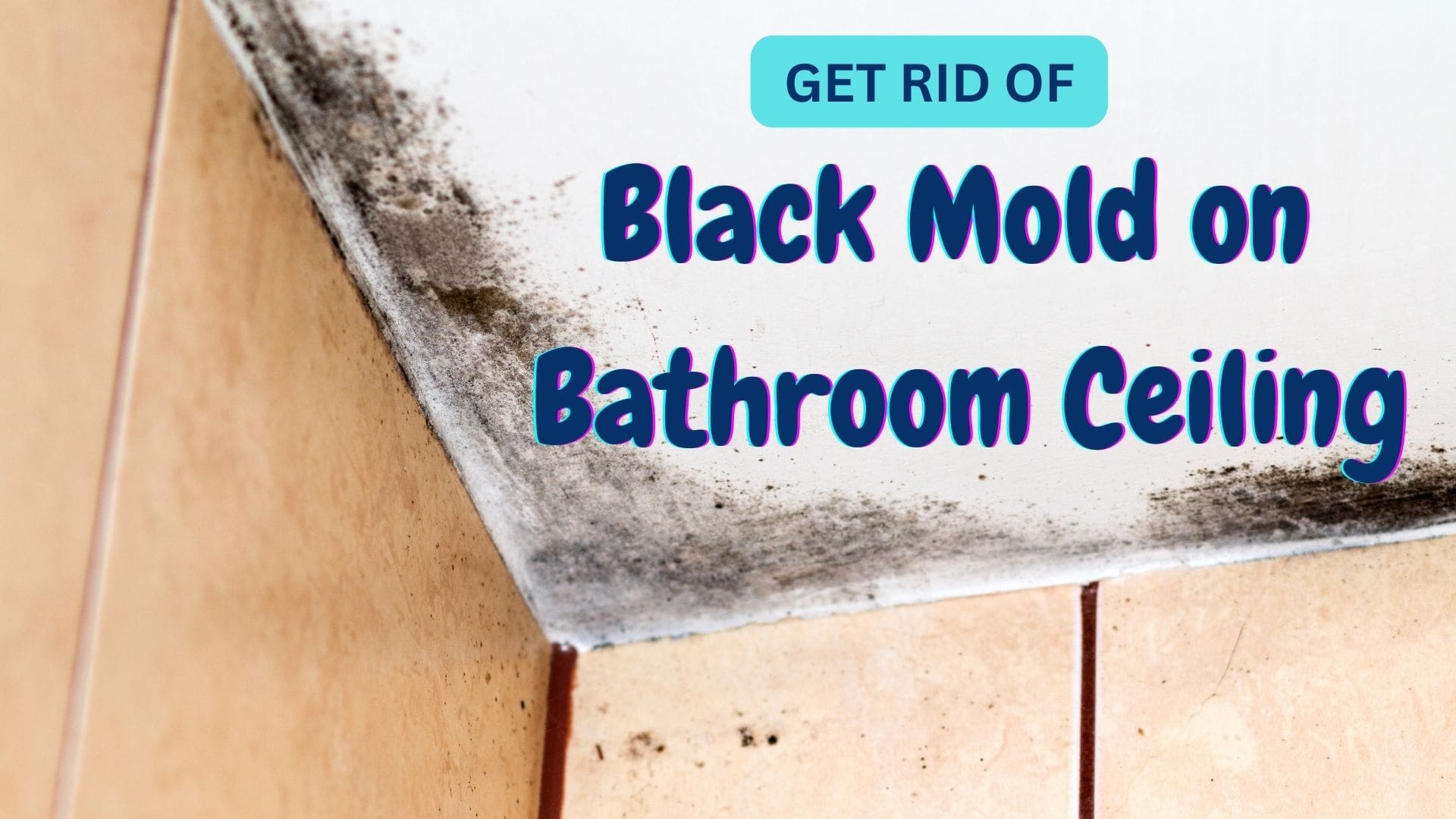The image is an advertisement or possibly a thumbnail for a DIY or help guide video on YouTube, emphasizing the removal of black mold from a bathroom ceiling. The main feature is a white ceiling heavily infested with black mold, particularly concentrated in the corners and spreading from left to right. The tiles on the wall underneath are salmon-colored, and there are tan-colored walls present on the left-hand side and bottom right corner. Additional mold spots appear minimally on the tiles, hinting at potential water damage above the ceiling. The top of the image features a teal background with blue text that reads "Get rid of black mold on bathroom ceiling." The advertisement does not specify if it promotes a product or service for mold removal. The image is devoid of people or any further instructions on resolving the mold issue.